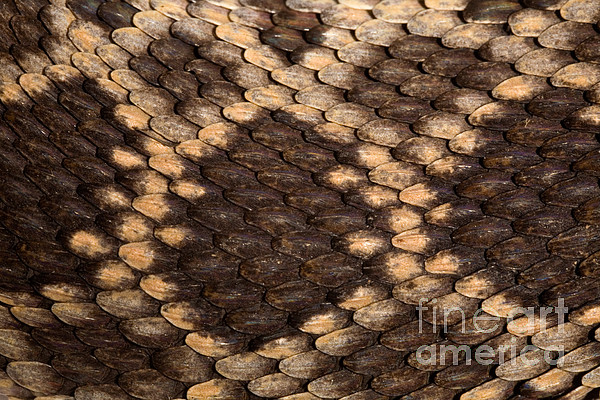This horizontal, close-up image vividly captures the detailed texture of reptile skin, most likely from a snake species resembling the diamondback rattler. The skin features a striking arrangement of scales or scutes, forming predominantly hexagonal and diamond-like patterns. These shapes are uneven, often smudged, and vary in size, with larger diamond shapes interspersed with smaller ones. The central dark brown scales contrast with the creamy pale brown edges, creating a visually intricate design. Towards the borders, especially in the lower right corner, there's a subtle watermark reading "Fine Art America," rendered in a ghostly, semi-transparent white font that blends softly into the image, almost as if reluctant to be seen. The overall effect evokes the impression of a meticulously woven fabric, with threads of brown and yellow creating a rich, textured pattern.